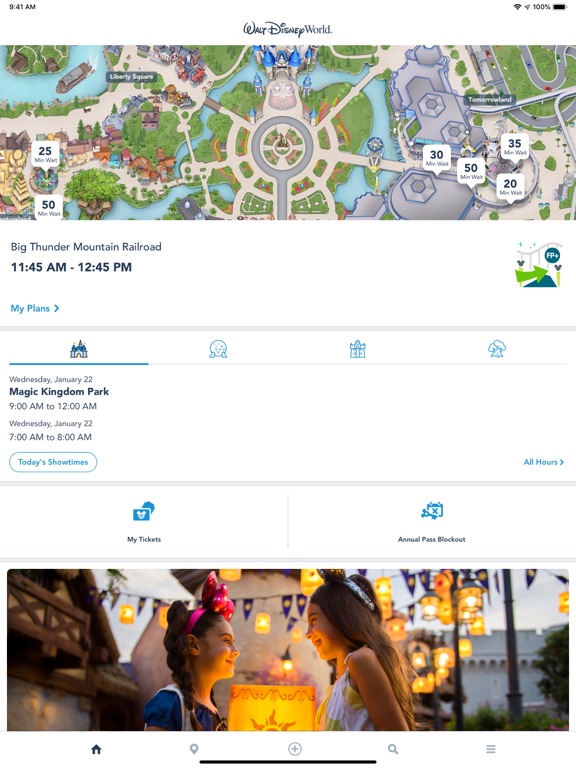This mobile screenshot showcases the Walt Disney World app, specifically focused on the Big Thunder Mountain Railroad Ride. The image captures a typical iOS device interface, indicated by the battery percentage, battery icon, and internet connection status in the top right corner, alongside the timestamp of 9:41 AM on the top left.

Central to the screenshot is an image of the Walt Disney World theme park with detailed ride information and wait times. Prominently highlighted is the Big Thunder Mountain Railroad Ride, available from 11:45 AM to 12:45 PM. The screen is titled "My Plans" and specifies that it is for Wednesday, January 22nd. It details the scheduling for Magic Kingdom Park, which operates from 9 AM to 12 AM on that date. Additionally, the screenshot lists "Today's Showtimes" from 7 AM to 8 AM.

Further sections within the app present various attractions in the Magic Kingdom Park, possibly including Liberty Square and Tomorrowland. Visible icons for "My Tickets" and "Annual Pass Blockout" are also included, along with promotional imagery.

Overall, this screenshot likely represents the personalized itinerary of a family vacation at Walt Disney World, meticulously planned to ensure a magical experience for the visitors.